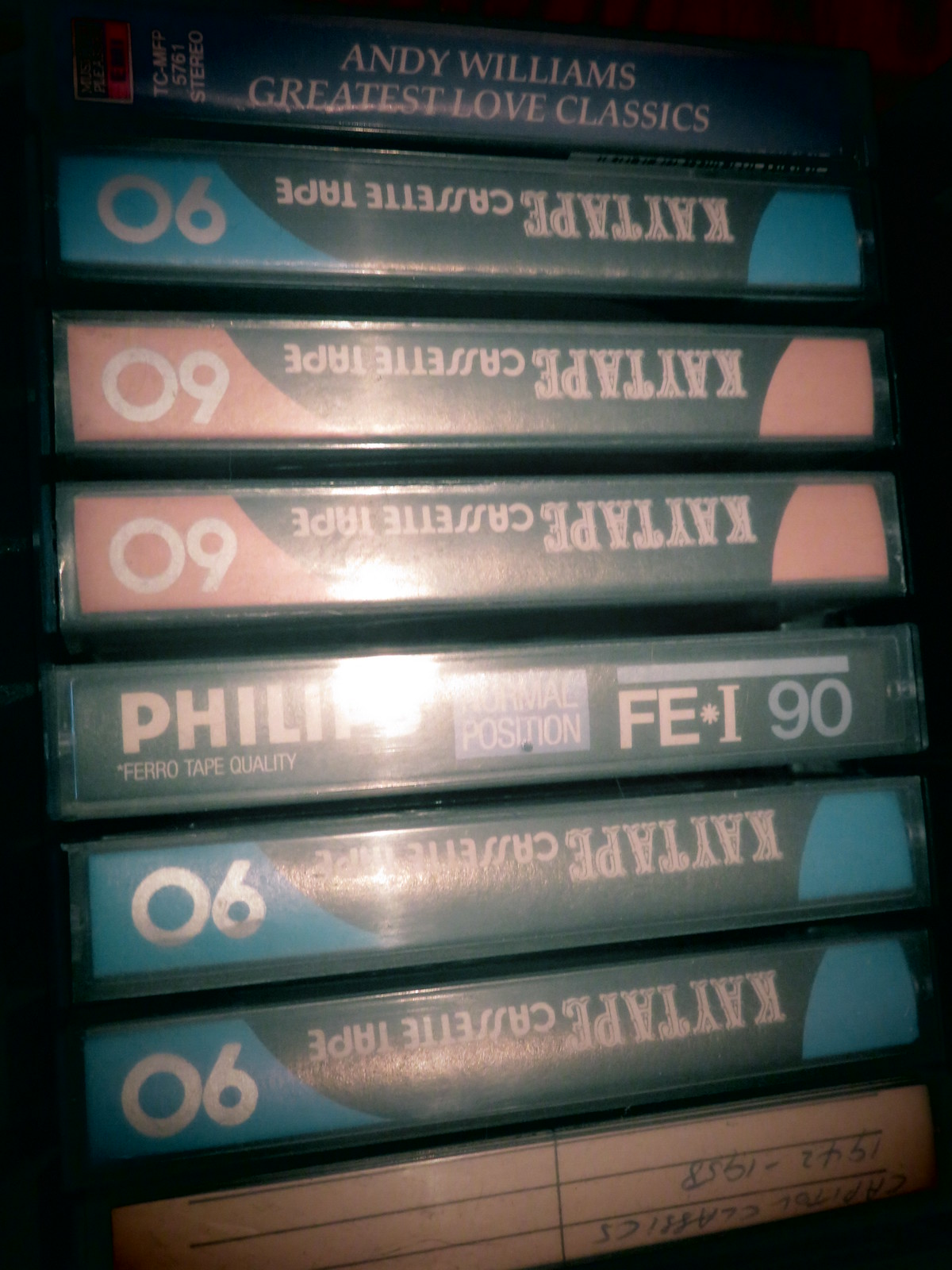In this digital indoor photo, the focus is on a series of stacked cassette tapes set against a completely black background. At the very top of the stack is a cassette in a blue case with white text that reads "Andy Williams Greatest Love Classics." Below it is a series of cassettes that are somewhat varied in their orientation. The second tape has blue edges with a black center and white upside-down text that reads "K-Tape Cassette Tape 90." Further down, there are two tapes with orange edges and black centers, both labeled "K-Tape Cassette Tape 60," also upside down. Following these tapes, there's a black cassette with part of the brand name "Philips" obscured by a bright flash, leaving visible blue and white text that includes "FEI 90." Beneath this are two more upside-down blue-edged cassettes similar to the ones mentioned above. At the bottom of the stack is a tape encased in a clear cover with a cream-colored insert, featuring illegible handwritten text in blue ink, which includes the dates "1942 - 1958." The tapes visually dominate the frame, contrasting sharply with the dark background that does not reveal any further details about the setting.